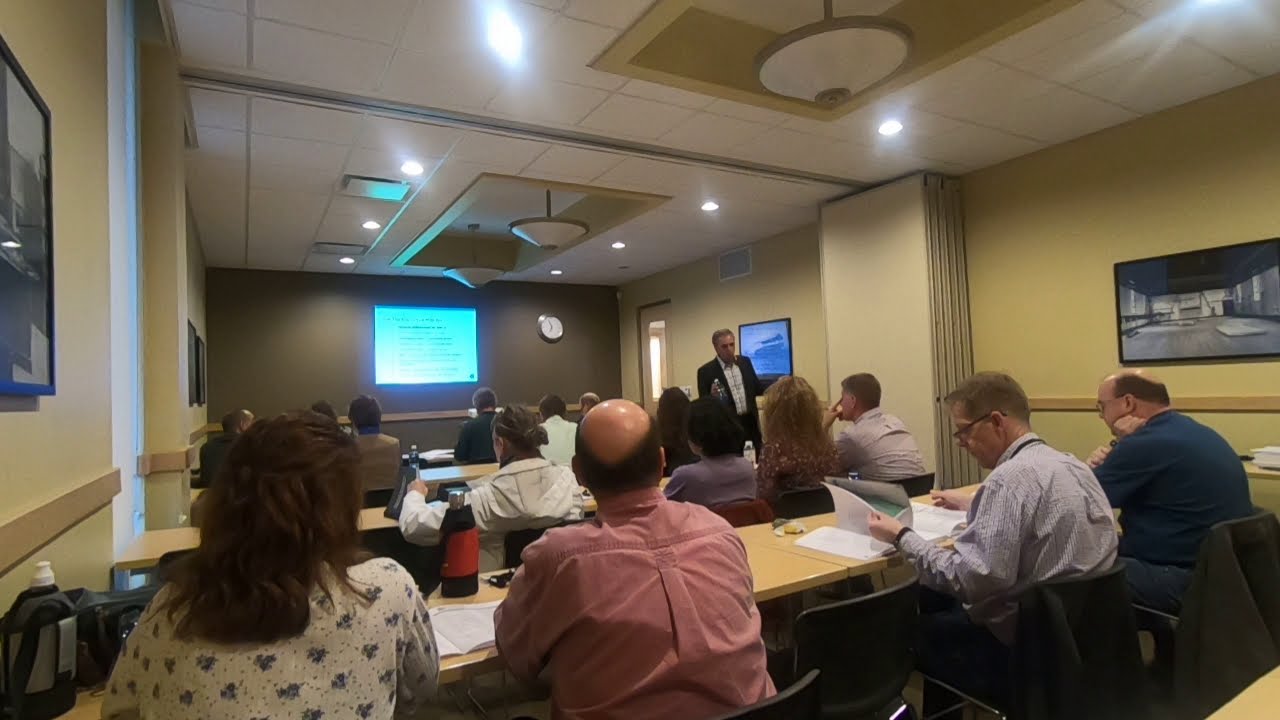The photograph captures a detailed scene of a conference or work-related meeting taking place in a professionally arranged room. The setting features rows of tables filled with approximately 20-25 attendees, both men and women, engaged in the proceedings. The participants, dressed in a range of casual office attire including collared shirts and varying hairstyles, are intently focused on an instructor. This instructor, a man clad in a suit and bow tie, appears to be delivering a PowerPoint presentation, moving around as he explains his points. A blue light emanates from the projector, casting a hue on the white, grid-style ceiling and illuminating a screen on the back wall. Surrounding this screen, which displays some text, is a variety of room decor including a white clock and multiple framed portraits hanging on the yellow and gray walls. The room is lit by several hanging lights positioned in different sections. Some attendees are taking notes on paperwork spread out before them, adding to the attentive atmosphere of this photographically captured professional environment.